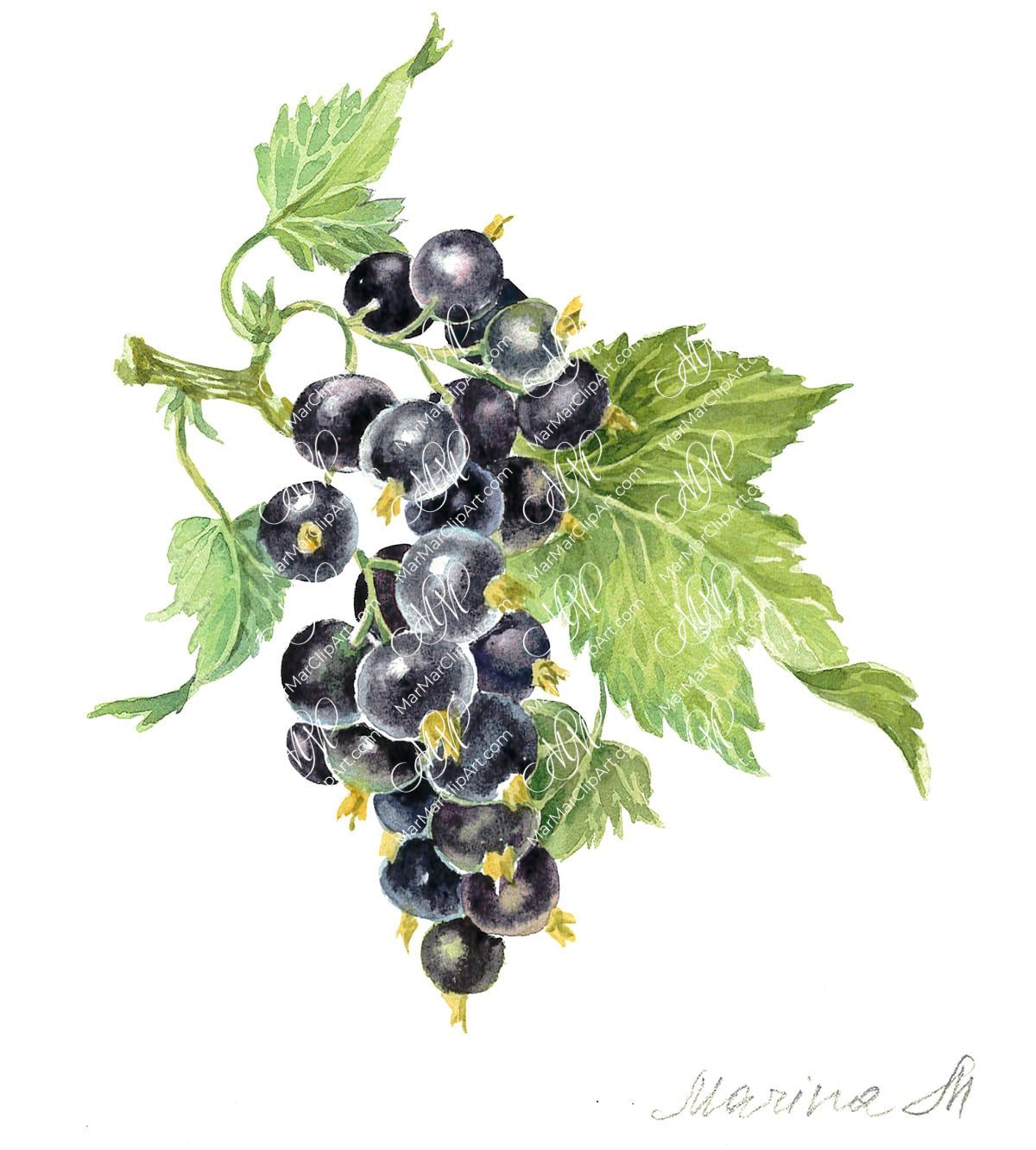The image is a detailed digitized artwork or watercolor painting that prominently displays a cluster of dark purple grapes on a green vine. The central focus is on the grapes, which are arranged densely together, with additional leaves extending to the left and right. The green leaves are detailed with white veins running through them. Each grape features a small, diagonal white imprint reading "M.A. Marked Morrow," indicating the artist or source. Additionally, a difficult-to-read signature, likely "Marina S.H.," appears at the bottom. The artistic piece captures the ripeness of the grapes, some tinged with a hint of yellow, set against the vibrant greenery of the vine and leaves.